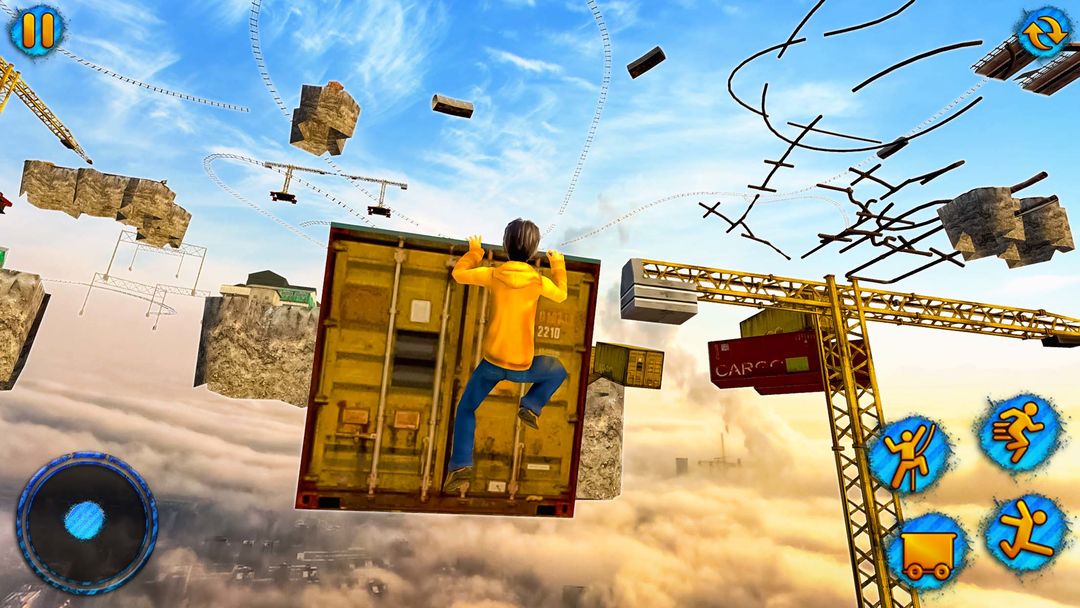In this avant-garde, fantastical artwork, the background features a deep, dark blue sky with wispy, white-striped clouds merging into gray and tan clouds at the base. The bottom half depicts a clearer blue sky with these thin clouds. The surreal landscape is cluttered with floating segments of massive stones or rocks, each square-shaped, and scattered pieces of cables and metal objects, including what resemble track lighting fixtures. Interspersed among these elements are shipping containers and cranes that appear to be lifting them, reminiscent of those used at dockyards.

Dominating the center of the piece is a man, seen from behind, climbing over what looks like the back doors of a shipping container. He wears a yellow long-sleeved hoodie, blue jeans, and brown shoes. His brown, shoulder-length hair sways as he ascends this free-floating door. To the man's right is a crane, with a vertical boom balanced by a horizontal arm and weights, enhancing the whimsical, gravity-defying nature of the scene.

In the bottom right corner, four yellow circles feature silhouettes of figures engaged in various activities—climbing, running, and jumping—adding to the dynamic, action-filled vibe. Additionally, there is a blue orb in the bottom left with the image of an old-school mining cart in yellow, next to a tan steel girder. Below all this surreal aerial display lies a dystopian cityscape, barely visible through a thick layer of smog, grounding the otherwise otherworldly scene in a touch of gritty realism.